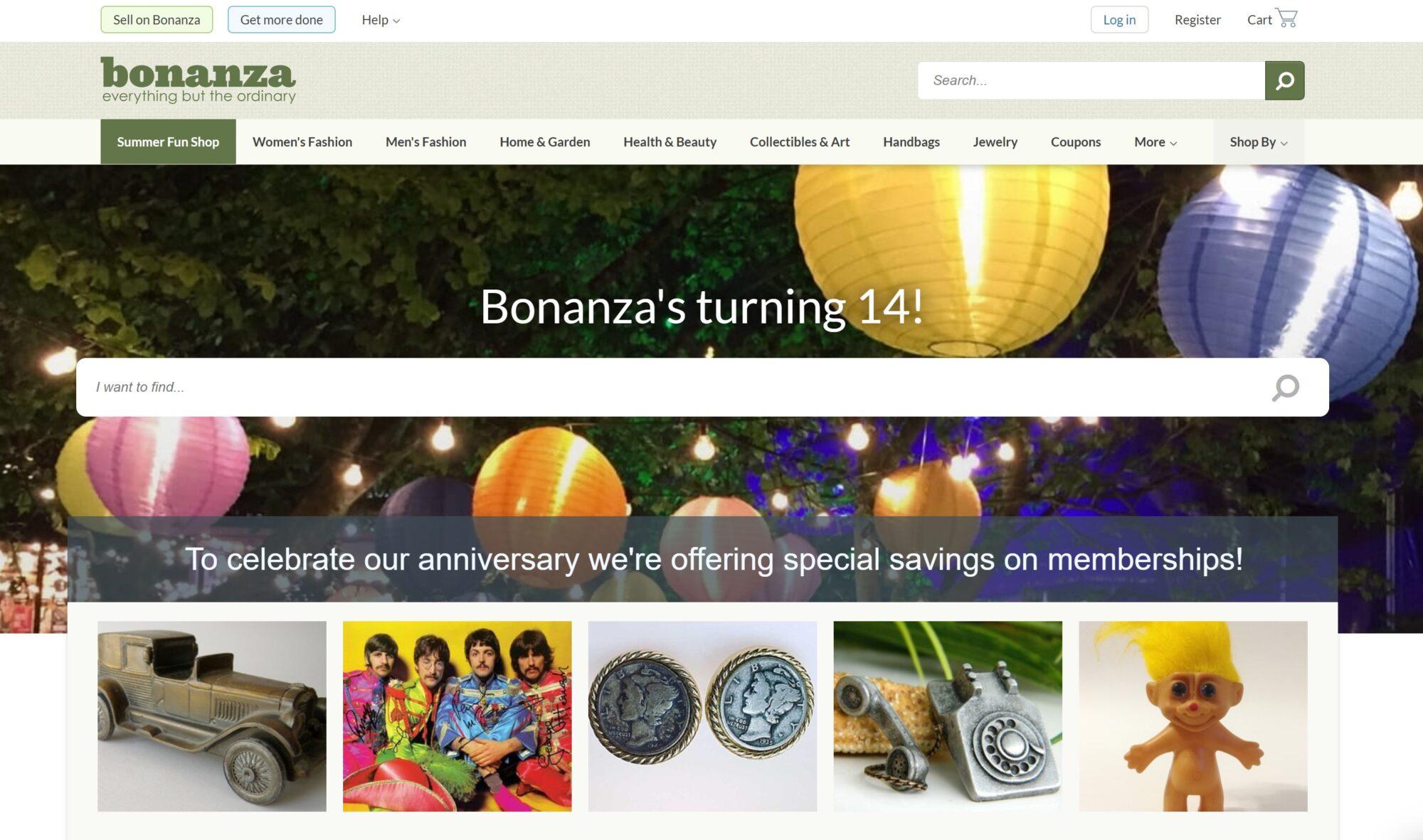On a clean white background, the upper portion of the image features two light gray buttons with black text that reads, "Sell on Bonanza" and "Get More Done." Adjacent to these buttons is a drop-down menu labeled "Help." On the right side, there's a "Log In" button followed by a "Register" button and a shopping cart icon.

The next section showcases a greenish-gray banner on the left, displaying the Bonanza logo and the slogan, "Everything but the ordinary." To the right, there's a white search bar accompanied by a green button with a white magnifying glass icon.

Beneath this banner, a green-highlighted segment features a blue background with white text that reads, "Summer Fun Shop." Below, in black text on a white background, are category labels: "Women's Fashion," "Men's Fashion," "Home and Garden," "Health and Beauty," "Collectibles and Art," "Handbags," "Jewelry," "Coupons," "More," and "Shop Buy."

The main visual depicts an outdoor setting adorned with colorful paper lanterns in shades of yellow, orange, pink, and purple. Dark green foliage forms the backdrop. Centered text in white announces, "Bonanza's Turning 14," alongside a search bar. Beneath, a pink banner with white text proclaims, "To celebrate our anniversary, we're offering special savings on memberships."

The bottom section includes five images: a toy car, a group of people looking forward, some old coins, an antique rotary phone, and an old, worn-out trowel with yellow bristles.